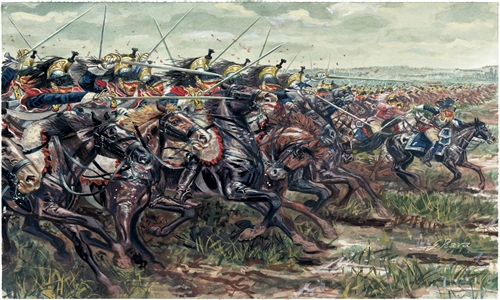This vibrant historical painting vividly captures the chaotic intensity of a battlefield scene, featuring a mounted cavalry charge amidst a tangle of soldiers and horses. The scene is dominated by a frenetic mêlée of saber- and sword-wielding soldiers, their expressions of fury and determination evident, with many pictured with open mouths likely unleashing ferocious battle cries. At the forefront are two commanding figures: one general in a striking red uniform blowing a bugle, while another in blue leads the charge. The intricacy of the horses' battle attire, possibly showcasing heraldry, adds to the richness of the scene. The painting, likely depicting European forces — perhaps Prussian — against a dark, ominous sky, realistically portrays the varied colors and types of the horses, the soldiers' black jackets with understated rain effects, and the terrain featuring both grass and sand. In the top right background, a valley or hill enhances the depth and setting of this dramatic piece.